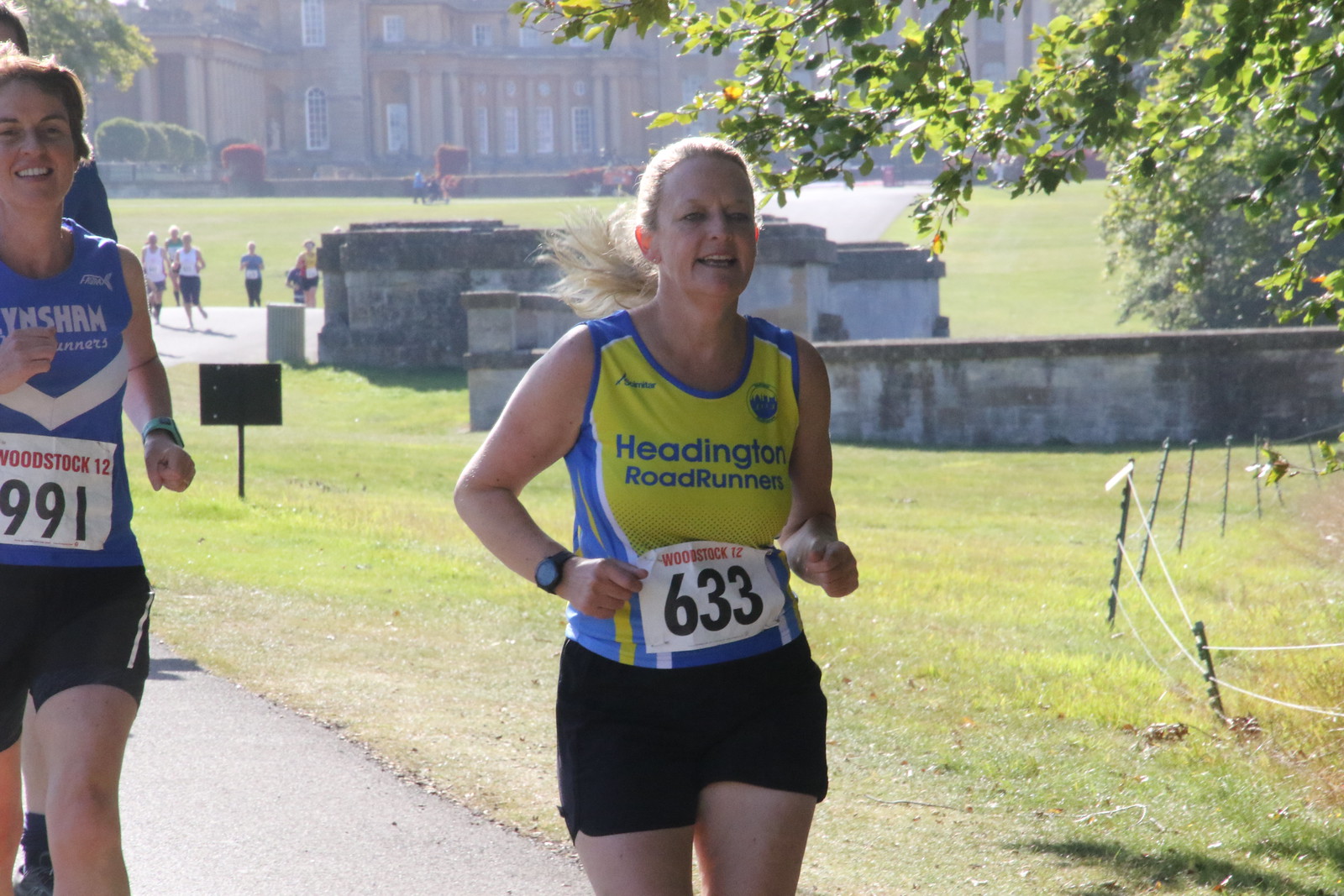The image captures a sunny day, likely during spring or summer, featuring a scene on what appears to be a college or university campus. The far background showcases a large, older building with several people visible in the distance. A green, grassy area is bisected by a wide asphalt walkway, and a stone wall meanders toward the foreground at various angles. In the mid-ground, runners can be seen making their way forward. The foreground prominently displays two women running towards the camera. The woman on the left, of European Caucasian descent, has short brown hair, a blue tank top with a white stripe just below her stomach, black shorts, and a race bib numbered 991 with the text "Woodstock 12" in red. Beside her and slightly ahead is another woman, also of European Caucasian descent, wearing a yellow tank top with blue sides that reads "Heddington Roadrunners." She has a race bib numbered 633, also featuring the text "Woodstock 12." Both women appear to be participating in a marathon or similar running event under a clear, bright sky.